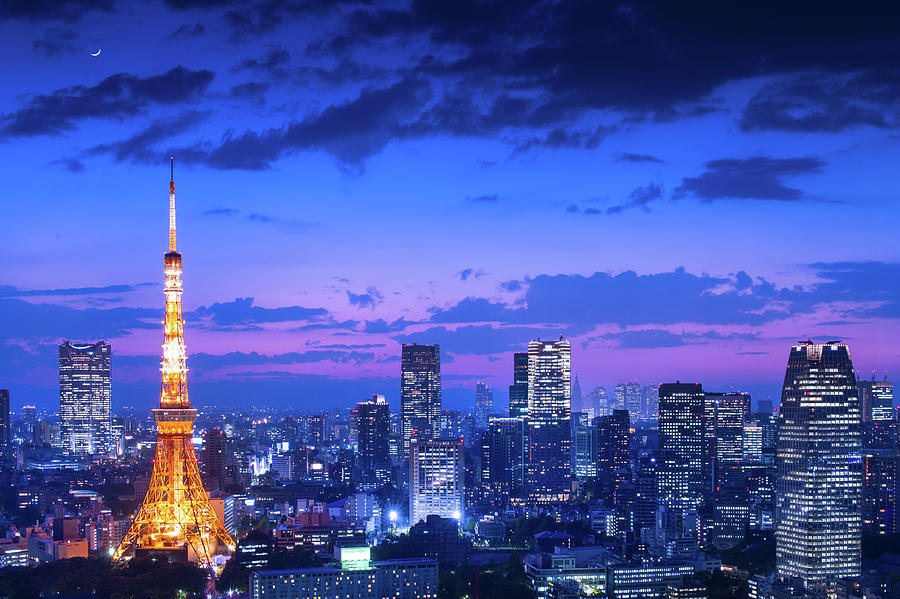The image is of a Paris cityscape at twilight, just after sunset, with the Eiffel Tower standing prominently on the left side, brilliantly illuminated in golden lights resembling a glowing needle. The scene features a mix of tall, rectangular skyscrapers adorned with numerous white lights. The sky transitions from a lighter blue near the horizon, tinged with pink and light purple hues, to a darker blue with a thick cluster of dark navy clouds in the upper right corner. A delicate white crescent moon is visible in the upper left corner, nestled within the deepening twilight. The overall ambiance captures the city as it shifts from evening to night, framed by the contrasting shades of blue and the lingering warmth of day.